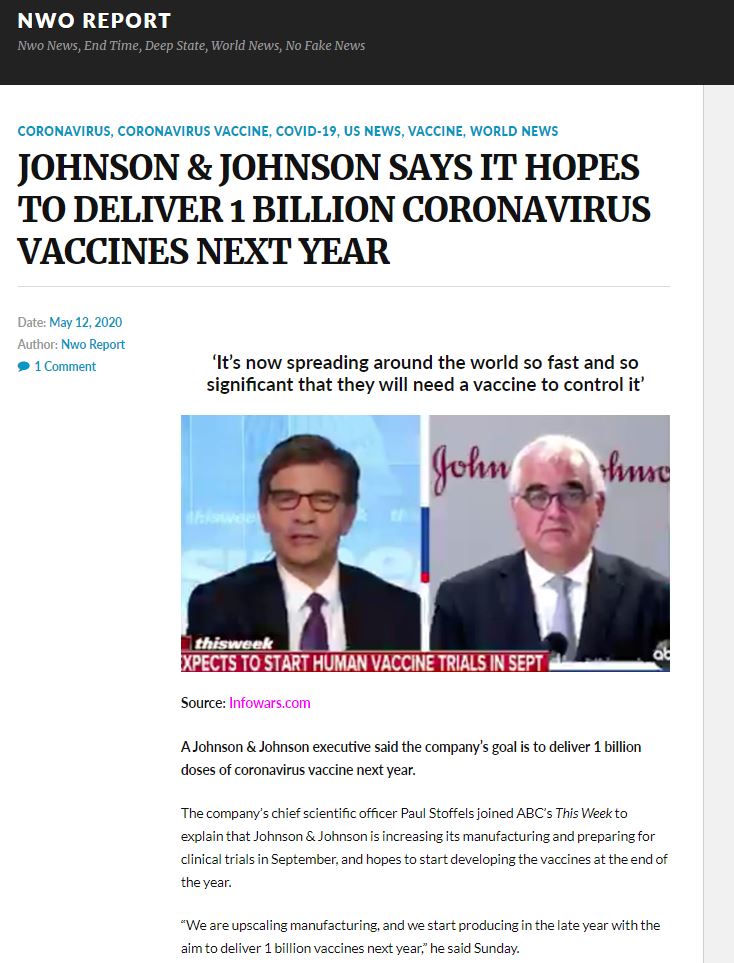This image is a screenshot from a mobile device displaying a webpage. At the top, there is a black header with white text indicating the site name: "NWO Report." This site is known for promoting conspiracy theories related to the "New World Order." Beneath the header, additional site information is provided: "NWO news, end time, deep state, world news, no fake news." Ironically, the disclaimer "no fake news" raises doubt about the site's credibility.

The main section of the page is set against a white background and lists several article tags including "coronavirus," "coronavirus vaccine," "COVID-19," "US news," "vaccine," and "world news."

Following the tags, the article title reads: "Johnson & Johnson says it hopes to deliver 1 billion coronavirus vaccines next year." A pull quote from the article states, "It's now spreading around the world so fast and so significant that they need a vaccine to control it." 

The article is accompanied by an image of George Stephanopoulos interviewing a Johnson & Johnson representative on an ABC news program. Notably, the article cites InfoWars.com, a well-known conspiracy theory website run by Alex Jones, as its source. The body of the article is displayed below the image.